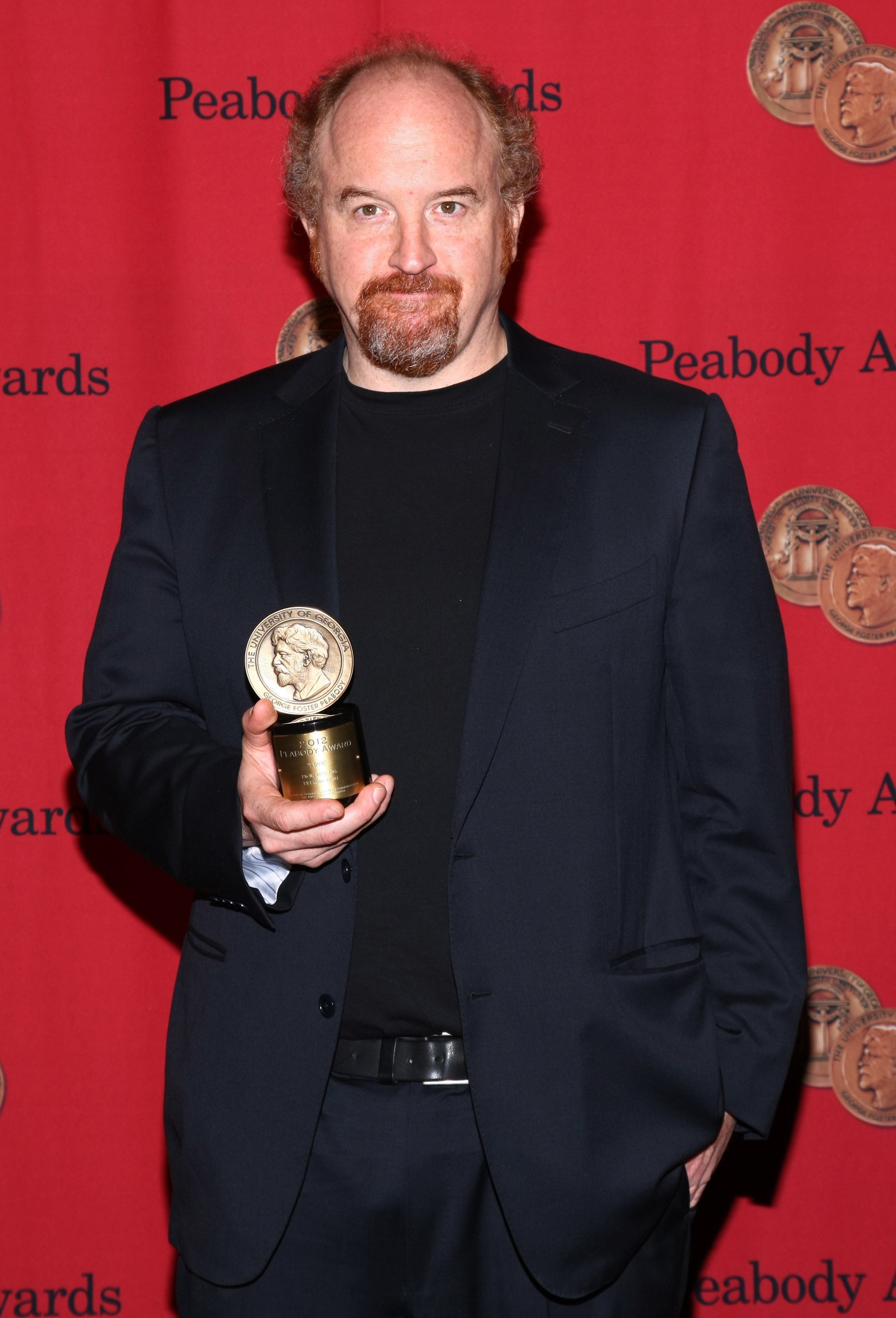In the photograph, a man is centrally positioned, facing forward. He is wearing a black suit coat over a black shirt, complemented by dark-colored pants and a black belt. The photo is cropped just above the knees. The man's left hand appears to be in his pocket, while his right hand is holding out a small statue with a rounded base and a coin-like top.

The man has very short, brownish-red hair that is balding on top with hair on the sides and sports a reddish mustache with a small reddish and gray beard. Behind him, the background is a red wall or curtain adorned with the words "Peabody Awards" repeatedly in black. The pattern also includes images of the award, depicted as coin-like objects, arranged periodically alongside the text. Some of the letters and images are partially obscured by the man standing in front.